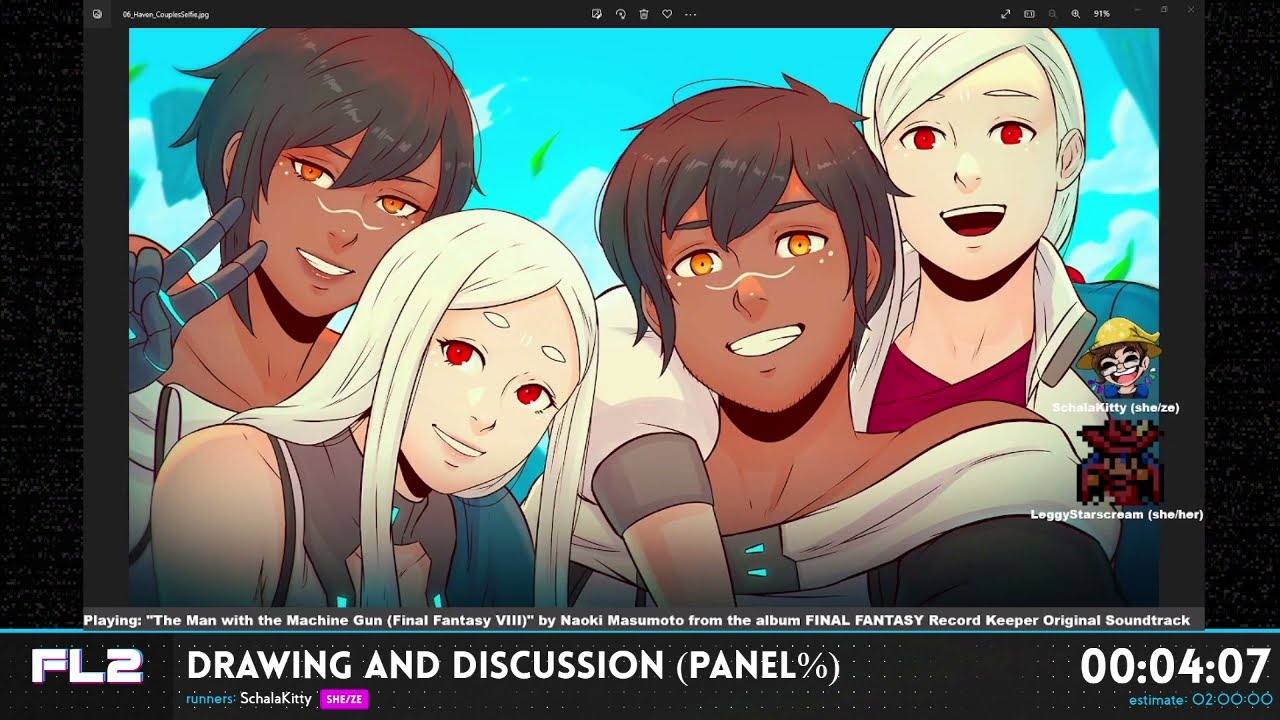The image showcases a well-drawn, colorful depiction of four anime-style cartoon characters, consisting of two males and two females. The characters are diverse in appearance, with two having blonde hair and red eyes, while the other two have dark hair and orange eyes. Their hair and outfits range in colors including browns, reds, tans, and turquoise. They are the focal point, spread across the forefront of the image against a turquoise background. Below the characters, text reads, "FL2 Drawing and Discussion Panel, Runners: Charlotte Kitty, She, Z," and "Percentage." Additionally, the screen mentions, "Playing 'The Man with the Machine Gun' from Final Fantasy VIII by Naoki Masumoto, from the album Final Fantasy Record Keeper Original Soundtrack." The overall setting appears to be from a tablet, possibly indicating a streaming app where this illustrated scene functions as the visual during music playback.